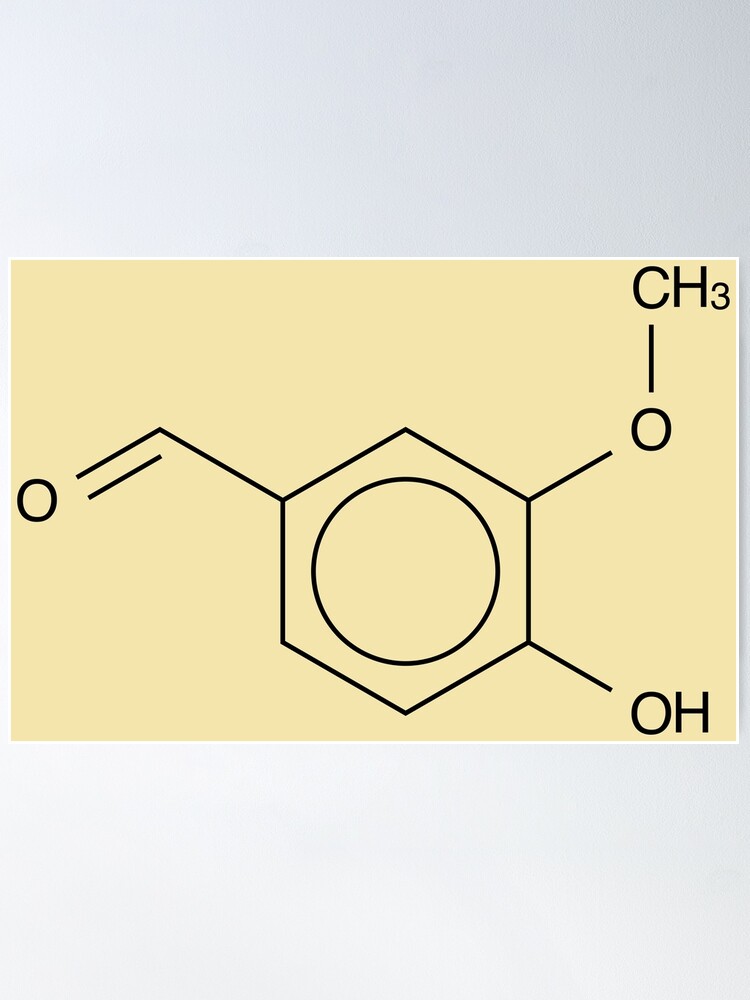The image showcases a detailed art print of a chemical compound on a rectangular card, centered on a textured white surface that gradients to a light gray in the upper right. The card features a thin white border with the main area filled in a saturated, yet muted, beige or cream color. Dominating the center of the card is a large hexagon outlined with black lines, with a smaller black circle inside. From various points of the hexagon, lines extend outward: one to a circle labeled "O" on the left, another to a circle labeled "O" just below "CH3" at the top right, and a final line pointing to "OH" at the bottom right. The hexagon, focal in the composition, serves as the central structure around which the molecular details are organized. The precise detailing and clean design suggest a digitally created print, meticulously representing the chemical element.